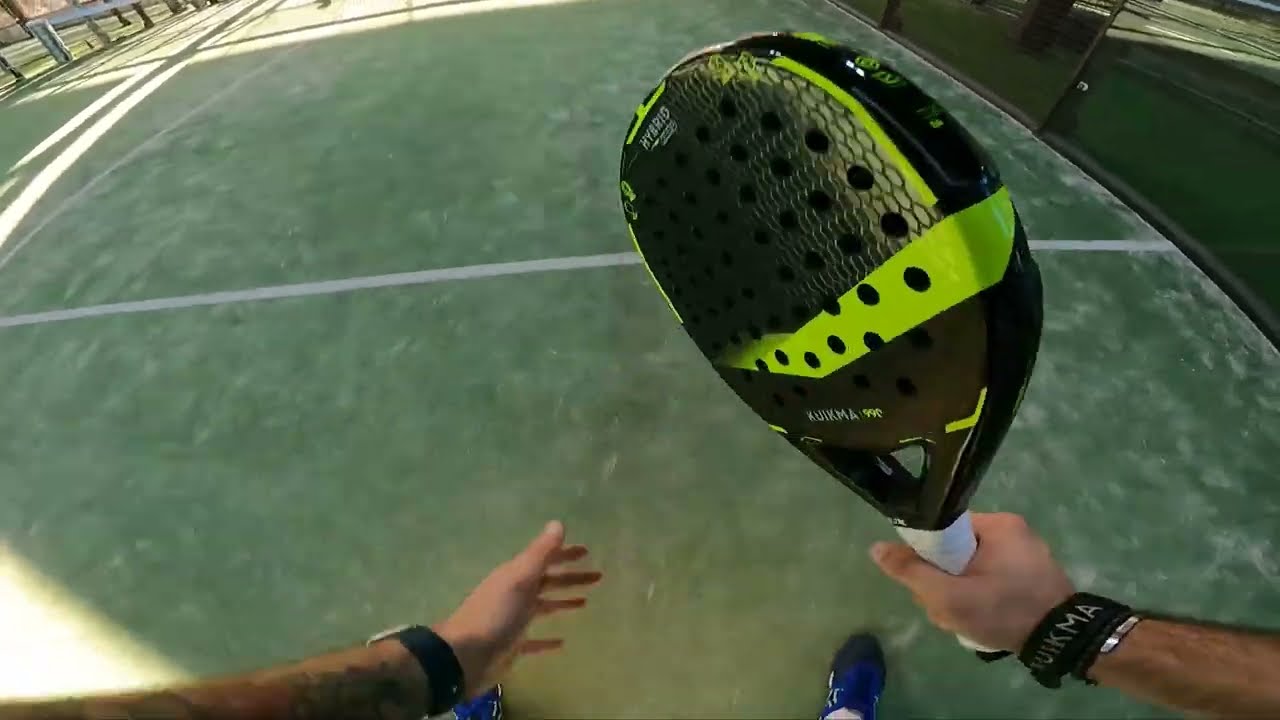In the image, a person is captured on an athletic court holding a Padel tennis racket with both hands. The racket, predominantly black with a light green streak running diagonally from the top-right to the bottom-left, features numerous tiny holes and a solid plastic cover on the visible side. Inscribed on it is “KUIKMA 99” along with a logo and the word “hybrid.” The grip of the racket is wrapped in white tape, and the person’s right hand, adorned with a black strap with white lettering and a silver bracelet behind it, is firmly grasping it.

The individual’s left hand, stretched slightly forward and downward, sports a wristwatch. Their blue shoe with a black toe cap extends forward on the ground. The surface of the court is green with white blotches and has white lines painted across it, one faint line running from the bottom left toward the top. The upper right corner of the image is darker, with light casting shadows on the ground.

This fisheye lens photograph accentuates the curvature of the scene, encompassing the court’s reflective glass on the right side. The overall setting suggests a versatile court, potentially repurposed for various racquet sports.